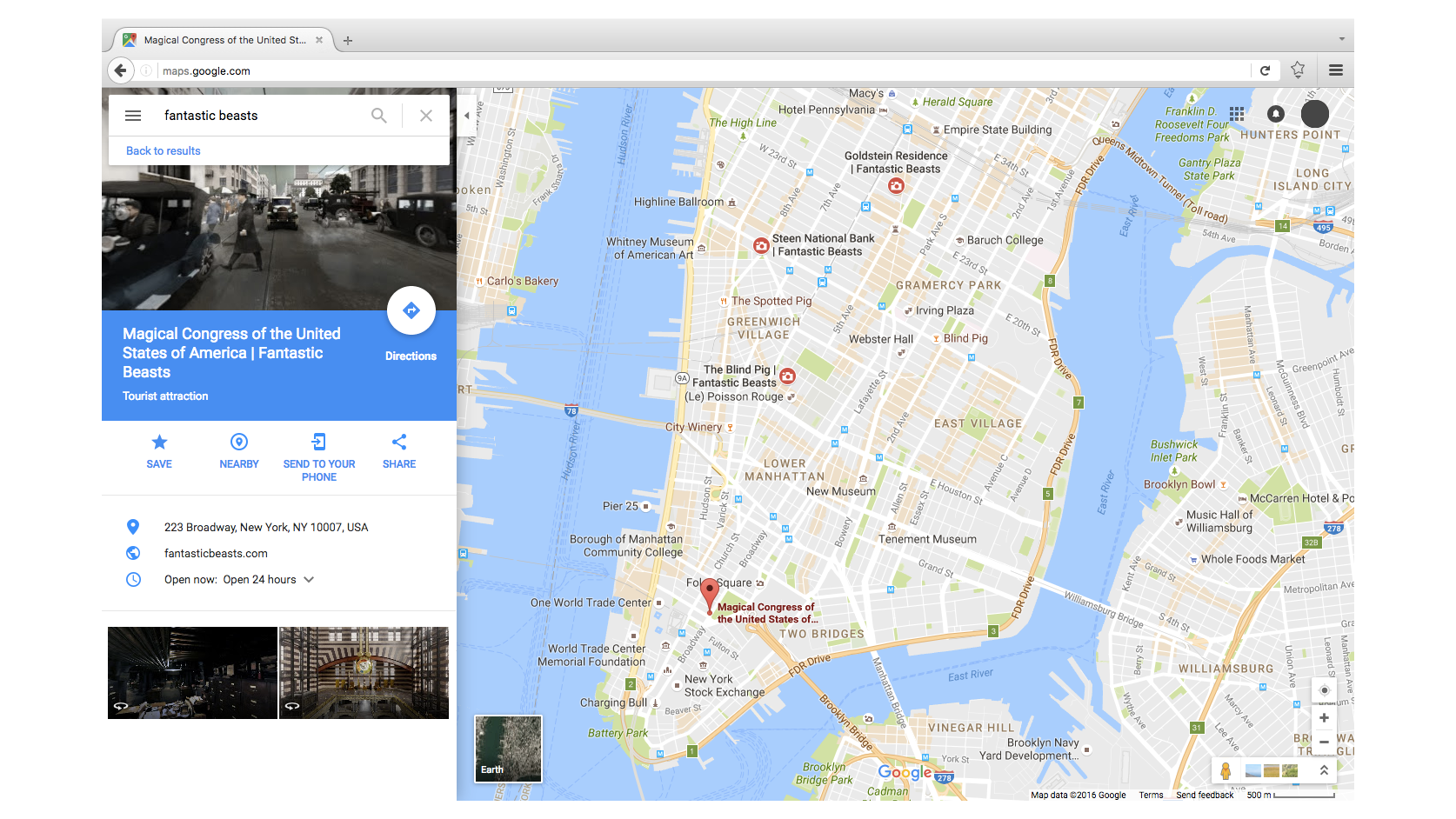The image depicts the Google Maps website. Dominating the right-hand side of the page is the interactive map itself, which features several location markers and pins. On the left-hand side, there is a detailed information panel. At the top of this panel is a search bar, where the user has entered the query "Fantastic Beasts." Directly below this, an image associated with the search result appears, labeled "Magical Congress of the United States of America, Fantastic Beasts." 

Next to this image, there is a "Directions" button, providing the option to navigate to the depicted location. Beneath this are four actionable buttons—Save, Nearby, Send to your phone, and Share—arranged side by side against a white background. Further down, the address of the location is listed as "223 Broadway, New York, New York 10007 USA." Additionally, a website for the location is provided: "fantasticbeasts.com."

Below the address, the operating hours are displayed, indicating that the place is currently open and operates 24 hours a day. At the very bottom of the panel, there is an overview section featuring various images of the location.